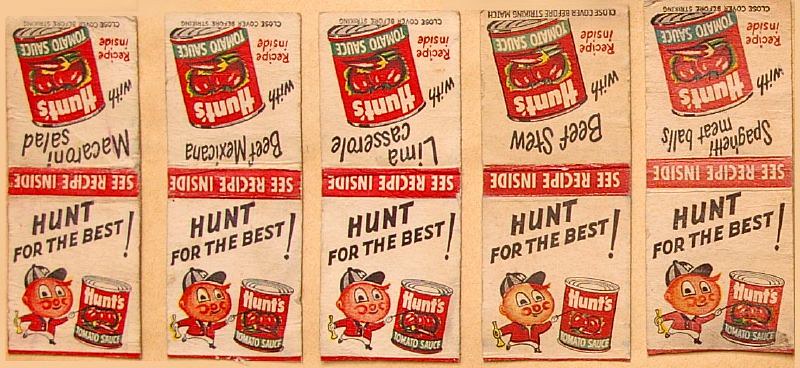This image showcases a collection of five vintage product labels for Hunt's Tomato Sauce, each vibrant and nostalgic in design. The labels prominently feature the slogan "Hunt for the Best," accompanied by a charming cartoon figure of a boy wearing a baseball cap. The boy is depicted holding a small trumpet, adding a whimsical touch to the labels. Each label is adorned with culinary suggestions, though the text appears upside down. The suggested dishes include: macaroni salad, beef Mexicana, lima casserole, beef stew, and spaghetti with meatballs. These labels capture the essence of a bygone era, when product packaging played a pivotal role in guiding home cooks' culinary adventures.